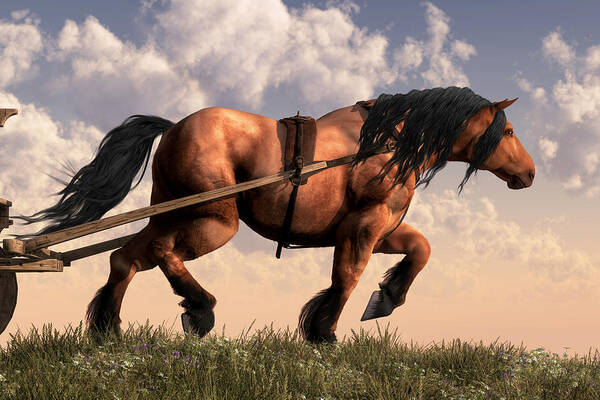This painting, reminiscent of a pre-rendered video game graphic, features a magnificent, muscular horse at the center. The horse, light brown in color, has a crimped, long black mane and tail, as well as long hair around its ankles. It is in mid-trot with its left front leg bent at the knee and lifted, and its back right hoof also off the ground, conveying a sense of dynamic motion. The horse is pulling a wooden cart, to which it is harnessed by a thin brown strap attached to two long wooden poles. Although most of the cart is out of the frame, a wheel is just visible on the left side of the image. The setting is a grassy area adorned with small white flowers, elevated against a dramatic sky that spans from the top to nearly the bottom of the picture, transitioning from a vibrant blue with scattered white clouds to a warm sunset hue.